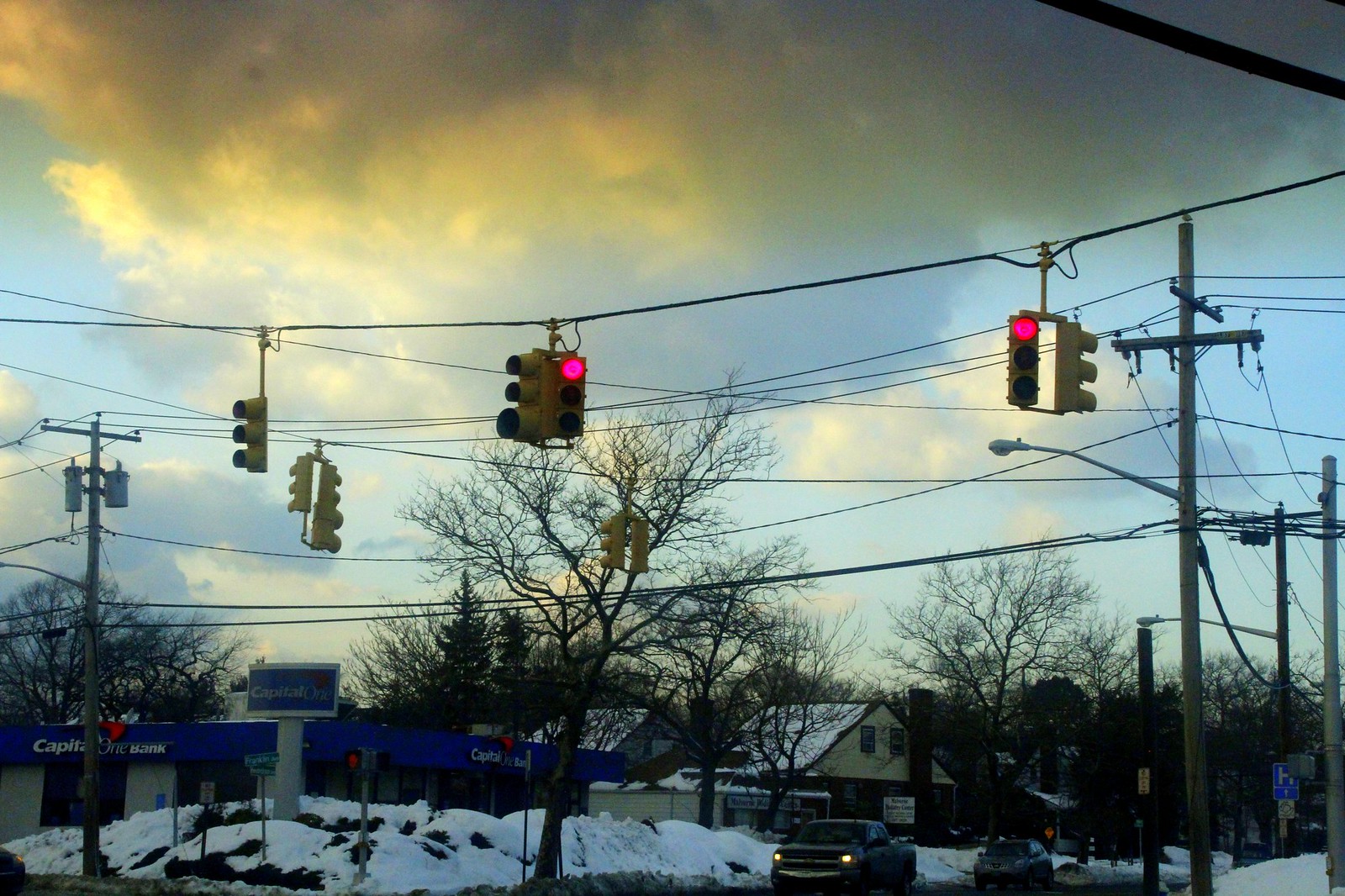The photograph, taken with a horizontally aligned rectangular frame, captures a striking scene at an intersection, viewed from an upward angle. The majority of the background is dominated by a densely clouded sky, painted in light blue hues. In the upper left quadrant of the frame, the clouds are subtly illuminated with a yellowish tint, suggesting the presence of sunlight breaking through.

At the bottom of the frame, there's a view of oncoming traffic, flanked by piled snow, indicative of a winter setting. Behind the vehicles, the landscape includes a couple of buildings, partially concealed by barren trees, their leafless branches stark against the sky.

Stretching horizontally across the center of the image are multiple electrical wires, adding a complex web of lines to the scene. Prominent among these are the street traffic lights, all of which display a uniform red, indicating a stop signal for the oncoming traffic.

The composition intricately balances elements of nature, urban infrastructure, and the seasonal environment, crafting a detailed and evocative urban winter tableau.